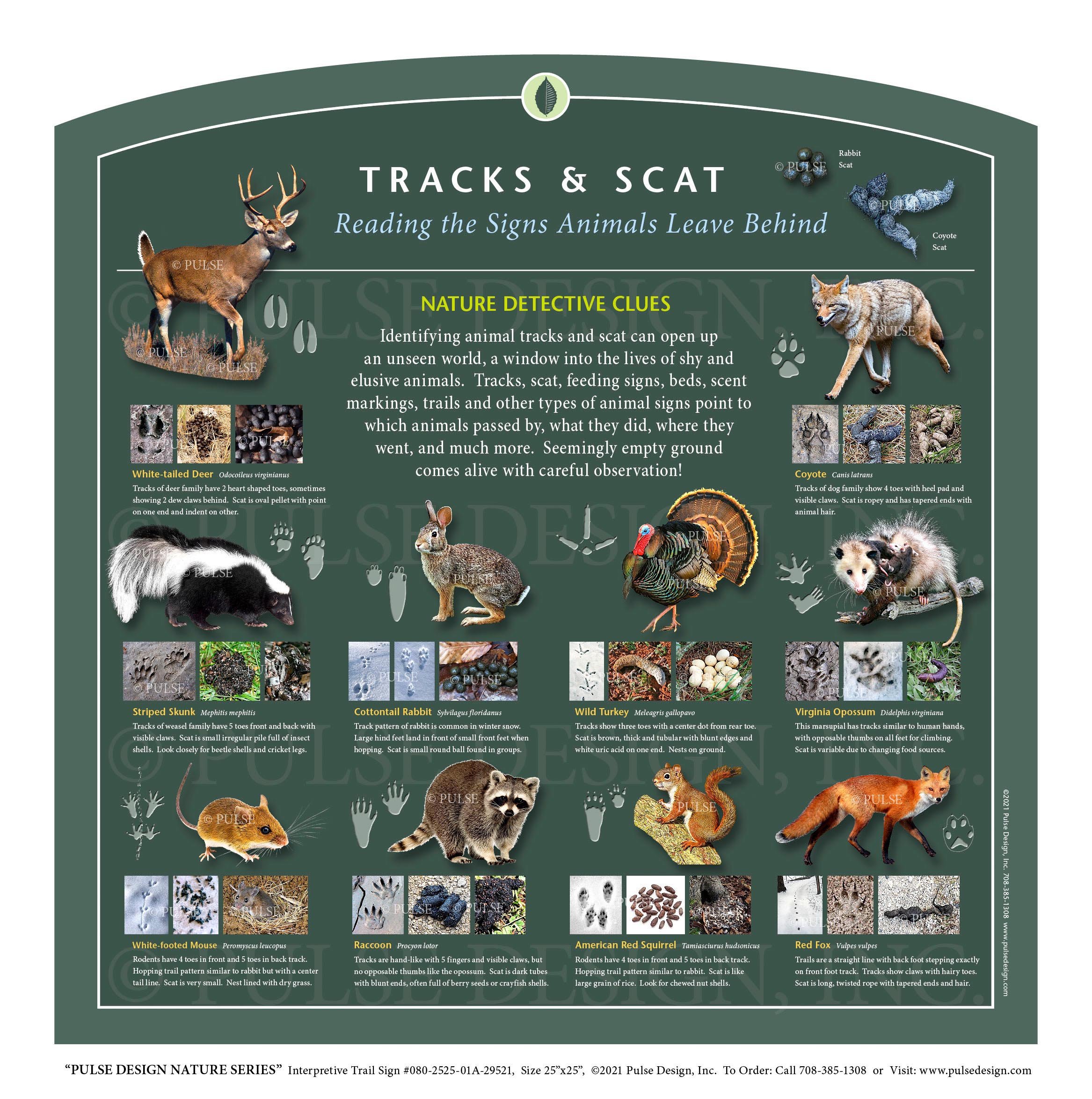This image features an educational sign with a dark green background, designed to help nature enthusiasts identify various wildlife through their tracks and scat. The sign is titled "Tracks and Scat: Reading the Signs Animals Leave Behind" in white lettering. Featured prominently are real photos of animals including a white-tailed deer, coyote, Virginia opossum, wild turkey, cottontail rabbit, striped skunk, white-footed mouse, raccoon, American red squirrel, and red fox. Each animal's photo is accompanied by illustrations of their tracks and multiple images of their scat in varying conditions, along with a small informative blurb. The educational value is enhanced by showing both visual and textual information on identifying these animals' presence in nature. At the bottom of the sign, it notes that it is part of the Pulse Design Nature Series Interpretive Trail Sign, with a website link to www.pulsedesign.com.